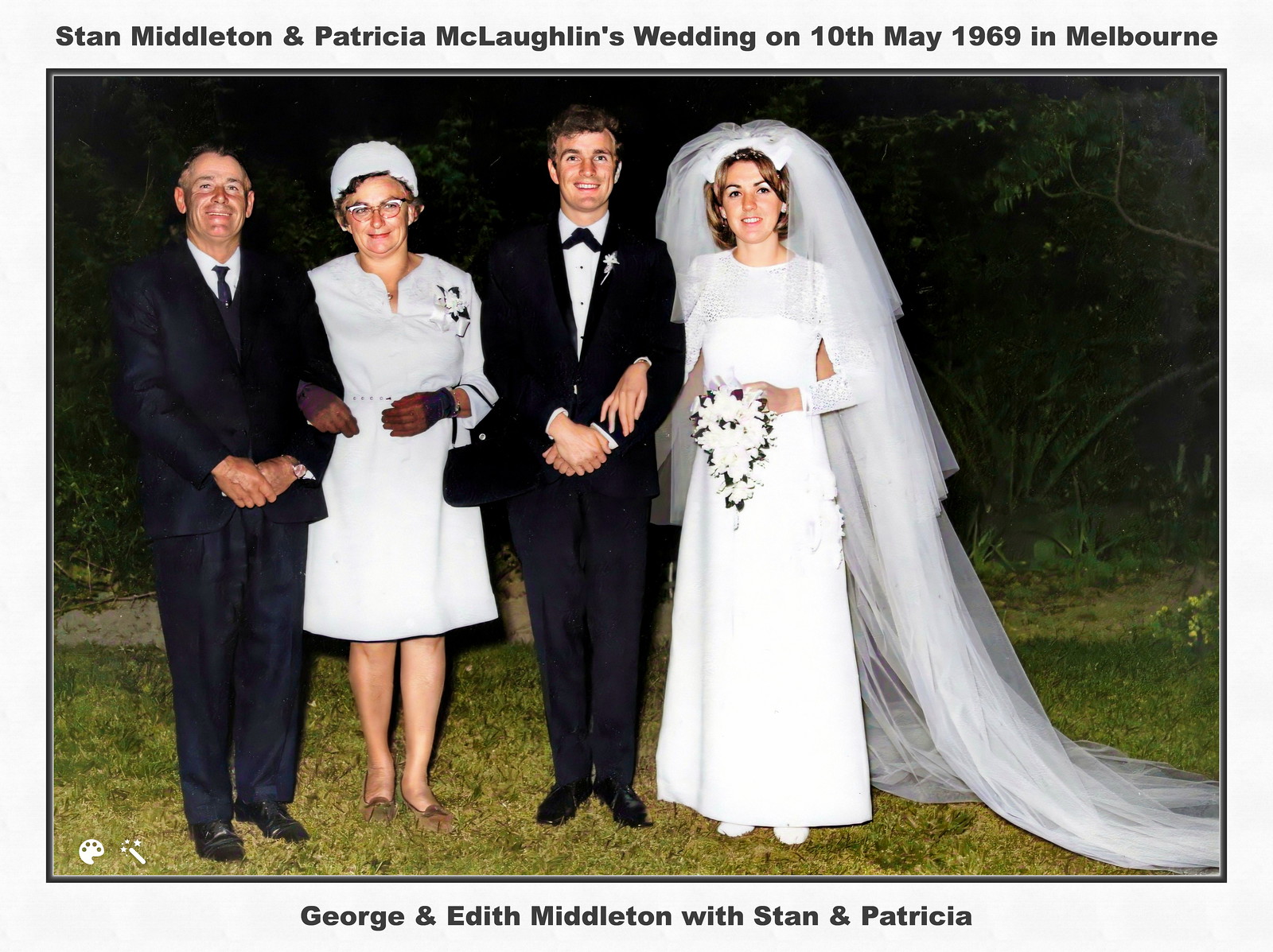This detailed color photograph in landscape orientation captures a vintage moment at a wedding, set against a slightly larger light gray background. A black headline across the top reads, "Stan Middleton and Patricia McLaughlin's Wedding on 10 May 1969 in Melbourne," and a black caption underneath identifies the subjects as, "George and Edith Middleton with Stan and Patricia." The photograph features four smiling individuals standing side by side on a grass field, facing the viewer.

On the right side stands the bride, Patricia, adorned in a long white veil and elegant white gown, holding white flowers at her waist. She has brown hair and is beaming with joy. Next to her is the groom, Stan, dressed in a classic black tuxedo with a white shirt, a black tie, and a flower lapel; he too is smiling brightly.

To Stan's right is a parent, Edith, wearing a chic white formal dress with a matching hat, dark gloves, and holding a black purse. Her attire is complemented by brown shoes and narrow glasses. Her arm is linked with that of George, standing on the far left. George, characterized by his black hair, wears a dark suit with a white shirt, a dark tie, and narrow glasses, giving him a distinguished appearance.

The style of the image is a blend of vintage photography, photographic representationalism, realism, and graphic design, emphasizing the authenticity and timelessness of this joyous occasion from 1969.